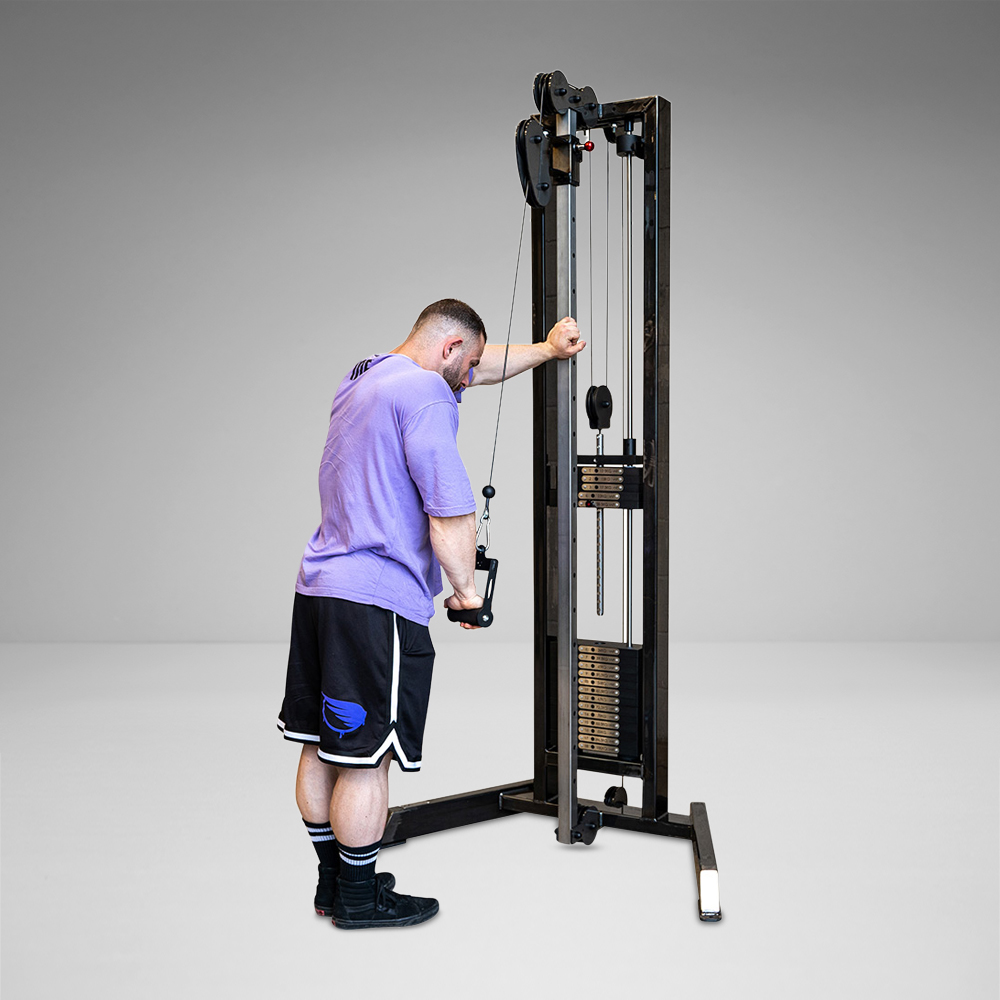This square photograph depicts a muscular Caucasian man working out on a black and silver weight machine in a stark white room with solid white floors and walls. The man sports a light purple t-shirt, black shorts adorned with white stripes along the sides and a blue design resembling an angel wing on the bottom right leg, black socks trimmed in white, and black tennis shoes. He is positioned with his back and left arm braced against the machine, and his right arm actively pulling down on a lever attached to the weights. His haircut is closely cropped with a fade, and he has a scruffy beard. The machine is a tall, upright model, designed with pulleys and wires to allow the lifting of various weights, suggesting a versatile range of workouts compatible with the equipment. The scene reflects a typical gym setting, focused on the intensity and precision of the workout.